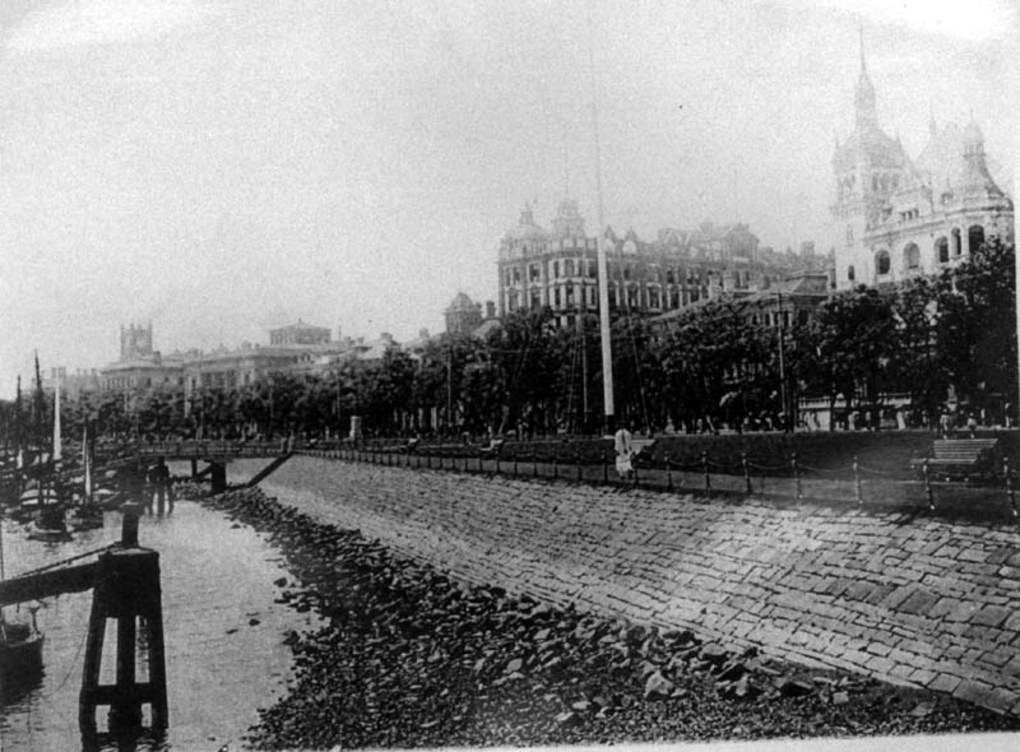This black and white image, grainy in some spots, captures an old European town's waterfront vista. The scene is dominated by a stone wall that slopes up to a spacious walkway, adorned with benches and a chain fence running along the top edge of the wall. Along the left-hand side sits a dock, bordered by sailboats, with a noticeable buoy floating in the water nearby. A wooden bridge extends from this dock to the town's walkway. In the foreground, a prominent white flagpole stands tall. The backdrop includes a mix of old buildings, one with a dome in the upper right corner and another to its left featuring two domes. Further to the right, there's a row of tall, dark trees cutting across the scene horizontally, under a white, grainy sky. The entire setting evokes a sense of timeless tranquility by the water.